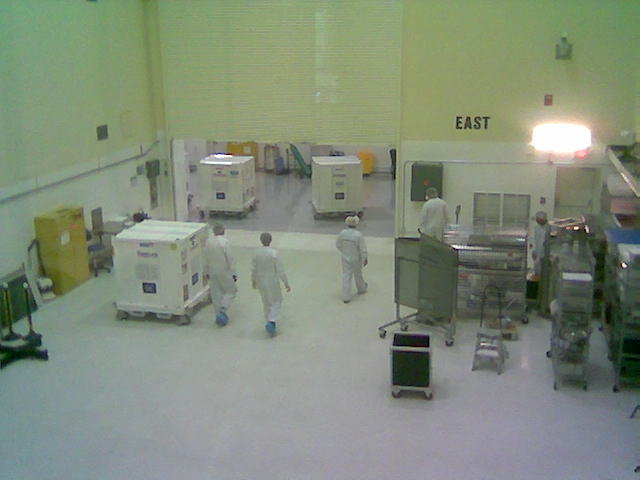The color photograph, taken from an elevated vantage point, captures the interior of what appears to be a sterile laboratory or warehouse environment. The rectangular image, approximately four inches tall by five inches wide, depicts a room with stark white flooring and predominantly white walls, transitioning to yellow on the upper half. Bold black lettering spelling "EAST" is prominently displayed on the back wall, accompanied by a bright white light to its right. Below the sign, metal shelving on wheels holds indistinct dark gray items. The room features large white boxes on wheels, possibly five feet high by six feet wide, clustered on the left side. 

Five individuals, clad in white coveralls or hazmat suits, complete with blue foot coverings, white hairnets, and rubber gloves, are positioned in the space. They appear to be transporting the white containers, which have visible numbers on them, towards an adjoining room that opens up at about the center line of the picture, with no traditional doorway but an open bottom portion of the wall. The bright, sterile lighting and clutter-free environment underscore the meticulous cleanliness of the setting.